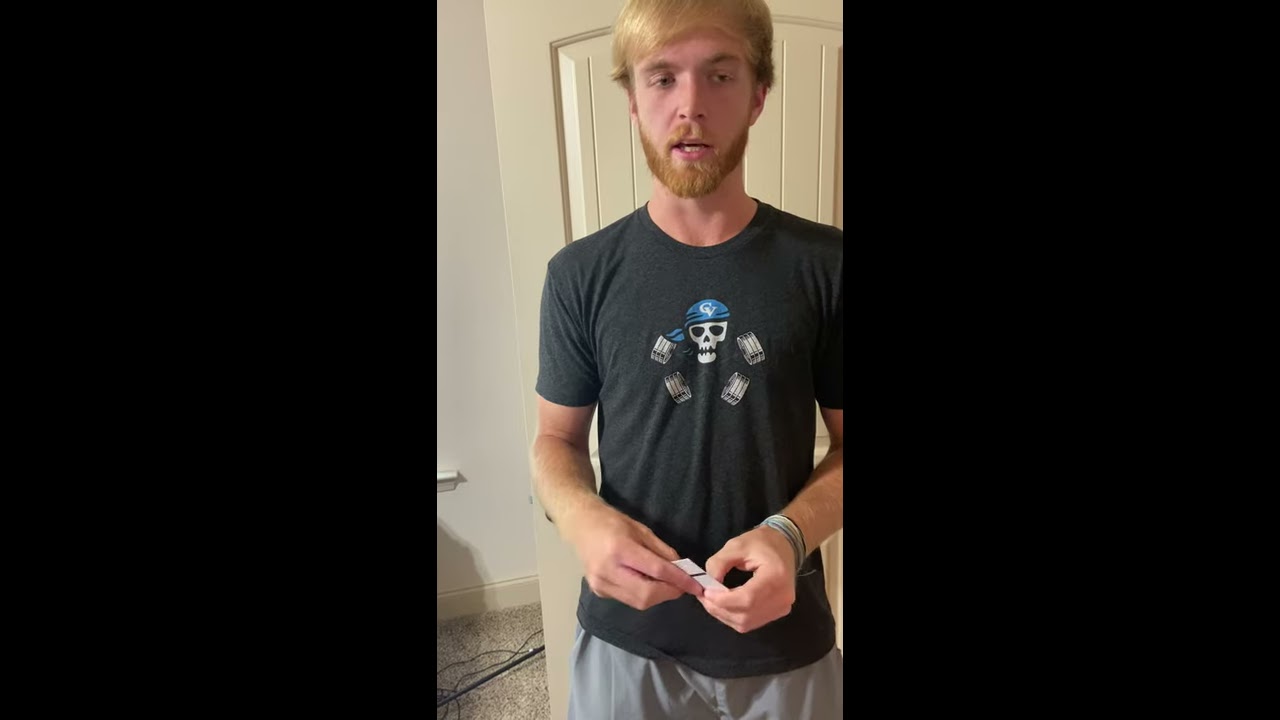The full-color, horizontally rectangular image is divided into three sections. The left and right sections are thick black panels, while the central panel features a young adult Caucasian male standing indoors. The man, appearing to be in his early 30s, has blonde hair that slightly covers his ears and a beard that is a mix of blonde and brown. He wears a dark heather gray short-sleeved t-shirt adorned with a white skull graphic. The skull is topped with a blue bandana featuring the letters "CV," and below it, two crossed barbells mimic a pirate flag design. The man also sports light gray pants and wristbands. He is holding a small piece of paper in his hands and is standing on a light beige carpet. The backdrop includes a white wall and an open, light buttercream-colored door. His body is facing the viewer, though he is gazing slightly to the right, with his mouth slightly open. Light from a window casts subtle shadows in the room, adding to the indoor ambiance.